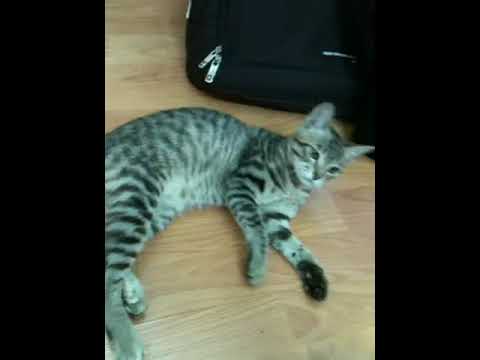The image, viewed within a vertical rectangular frame against thick black borders, showcases a small, gray and black striped cat lying on its left side on a light oak-colored wood floor. The photograph, taken with a cell phone, features the cat in the center, reaching up with its paw towards a human hand extending from the lower right corner. The hand, possibly a man's, is partially visible, adorned in a black sleeve, and positioned palm up. The interplay between the blurry hand and the cat's paw draws immediate focus. In the background, a black zippered bag, resembling a laptop case with silver zippers, partially appears, adding context to the setting. The overall style is one of photographic realism.